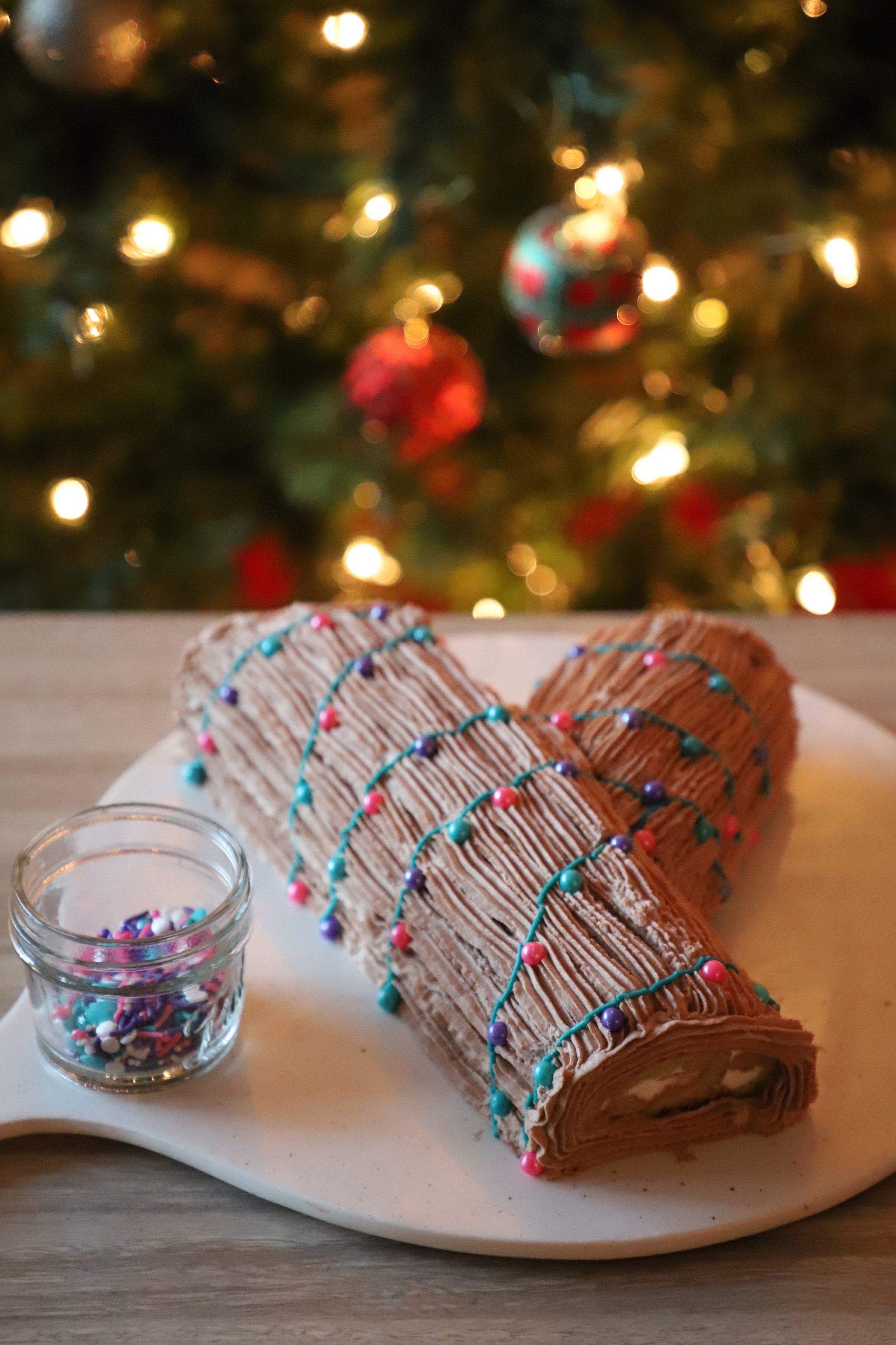This color photograph captures a festive holiday scene featuring a meticulously decorated chocolate yule log cake. The yule log cake, a classic Christmas tradition, is crafted from a chocolate sponge cake rolled into a log shape, adorned with brown frosting detailed with striations to mimic tree bark. In this image, there are actually two yule log cakes, crisscrossed atop a round platter with a handle, adding a rustic touch. The cakes are festooned with thin green frosting lines symbolizing electrical wiring, which are embellished with multicolored beads and sprinkles resembling Christmas lights, including shades of purple, green, pink, red, and blue. The interior of each log reveals a luscious white creamy filling. Accompanying the log cakes is a glass jar filled with similar decorative beads, placed on a light brown wooden table. The background showcases an out-of-focus Christmas tree adorned with green branches, red and green spherical ornaments, and twinkling white lights, encapsulating the festive spirit of the season.